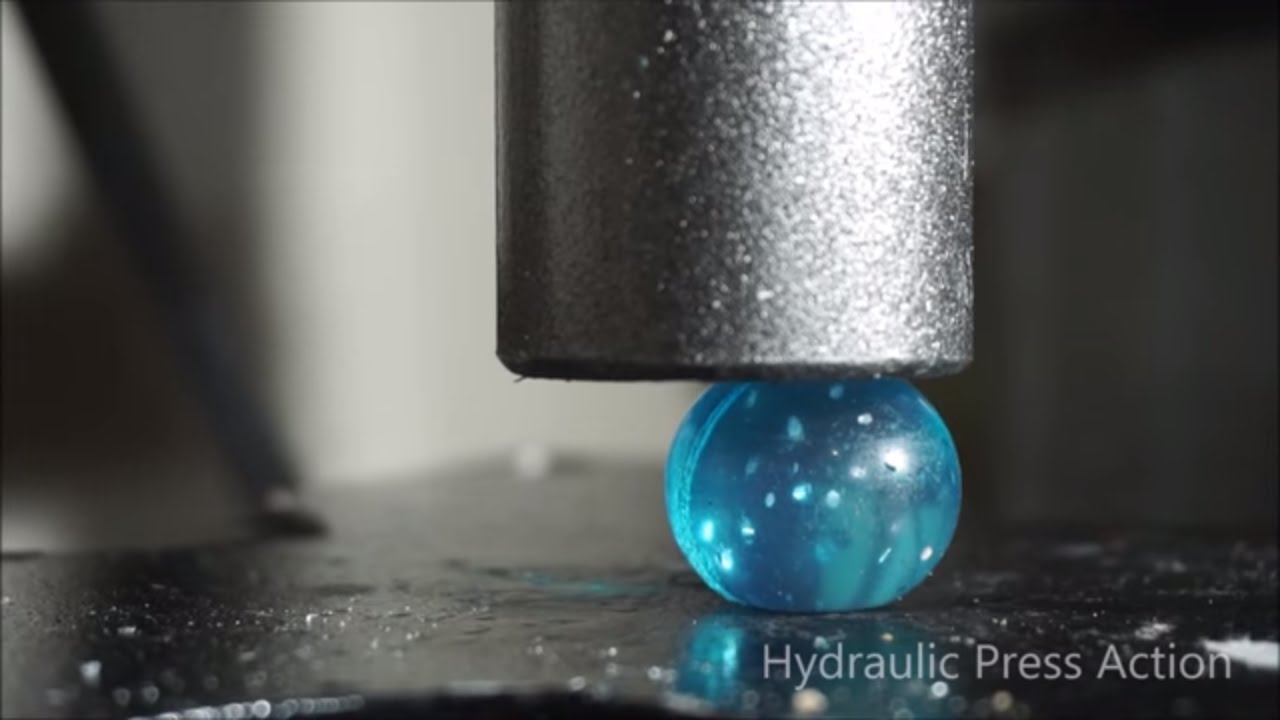The color photograph, captured in landscape orientation, focuses on a hydraulic press in mid-operation. The central object is a lustrous steel cylinder descending from the top of the image, halfway down and pressing onto a blue semi-transparent ball. Underneath the ball, the gleaming metal bed of the press is visible, scattered with gritty particles. The background is a complex mix of mechanical parts in grayscale tones, with a mysterious black object stretching across the rear. Closing details are provided by the text at the bottom right corner that states "Hydraulic Press Action," in bold white lettering. The depiction aligns with Photographic Representationalism, giving a realistic portrayal of the press in action.